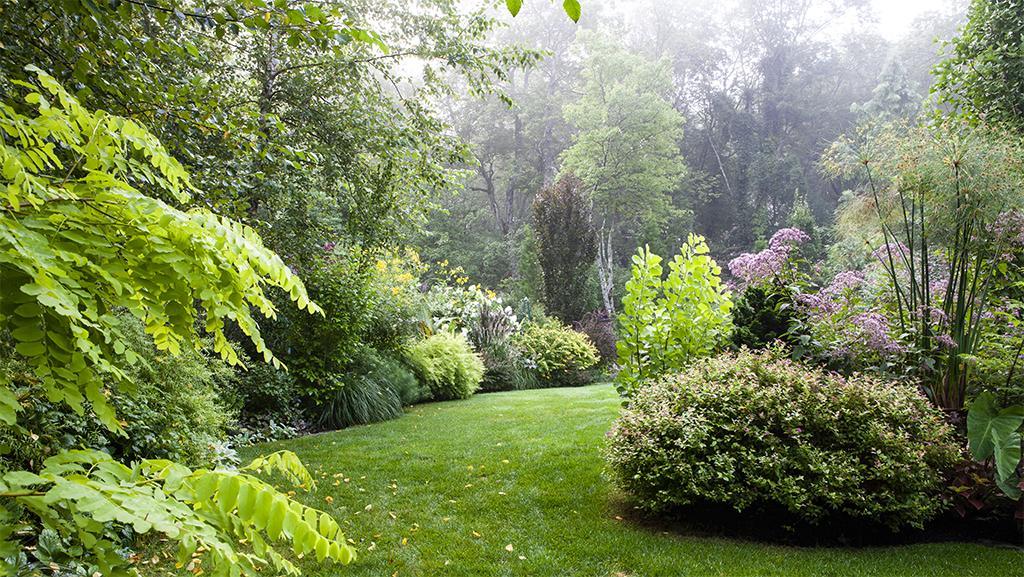This image showcases an expansive, well-manicured garden that exudes a peaceful and inviting atmosphere. The lawn, a verdant green path, gently curves into the distance, bordered by meticulously trimmed shrubs and lively vegetation. On the right side, a diverse array of shrubs, including a particularly large and neatly pruned one adorned with purple wildflowers, adds a splash of color. To the left, the scene is decorated with ferns close to the camera, giving way to more substantial trees further back. The entire garden is enclosed by tall, majestic trees, enhancing the secluded and tranquil feel of the space. The sky visible through the treetops appears slightly foggy or overcast, indicating a calm, temperate day. This serene, picturesque setting is likely part of a residential property, suggesting an affluent home due to the garden’s impeccable upkeep. The setting is ideal for outdoor activities such as running, walking pets, or simply enjoying a leisurely stroll, embodying both natural beauty and meticulous care.